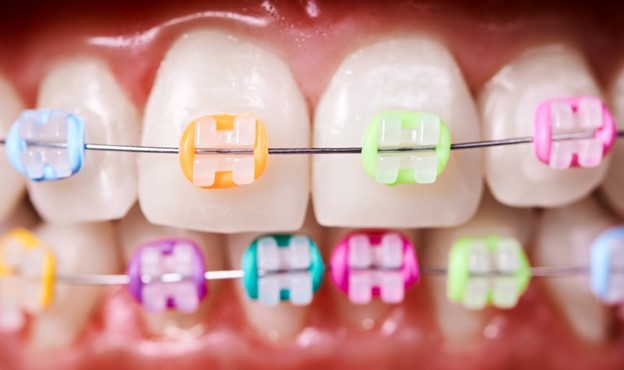This close-up photograph captures the inside of a person's mouth, focusing primarily on their teeth and gums adorned with braces. The image emphasizes the upper and lower sets of teeth, which are both fitted with braces that feature colorful rubber bands. On the upper row, the first four teeth sport an array of vibrant bands: blue, orange, light green, and pink. Below, the bottom teeth also display a dazzling selection with orange, purple, teal, magenta, light green, and light blue bands. The braces are connected by a central wire that threads through metal brackets affixed to each tooth. The overall image gives a detailed view of the orthodontic appliance and the colorful way the rubber bands are used to decorate the braces, although some parts of the lower teeth and braces appear slightly blurred.